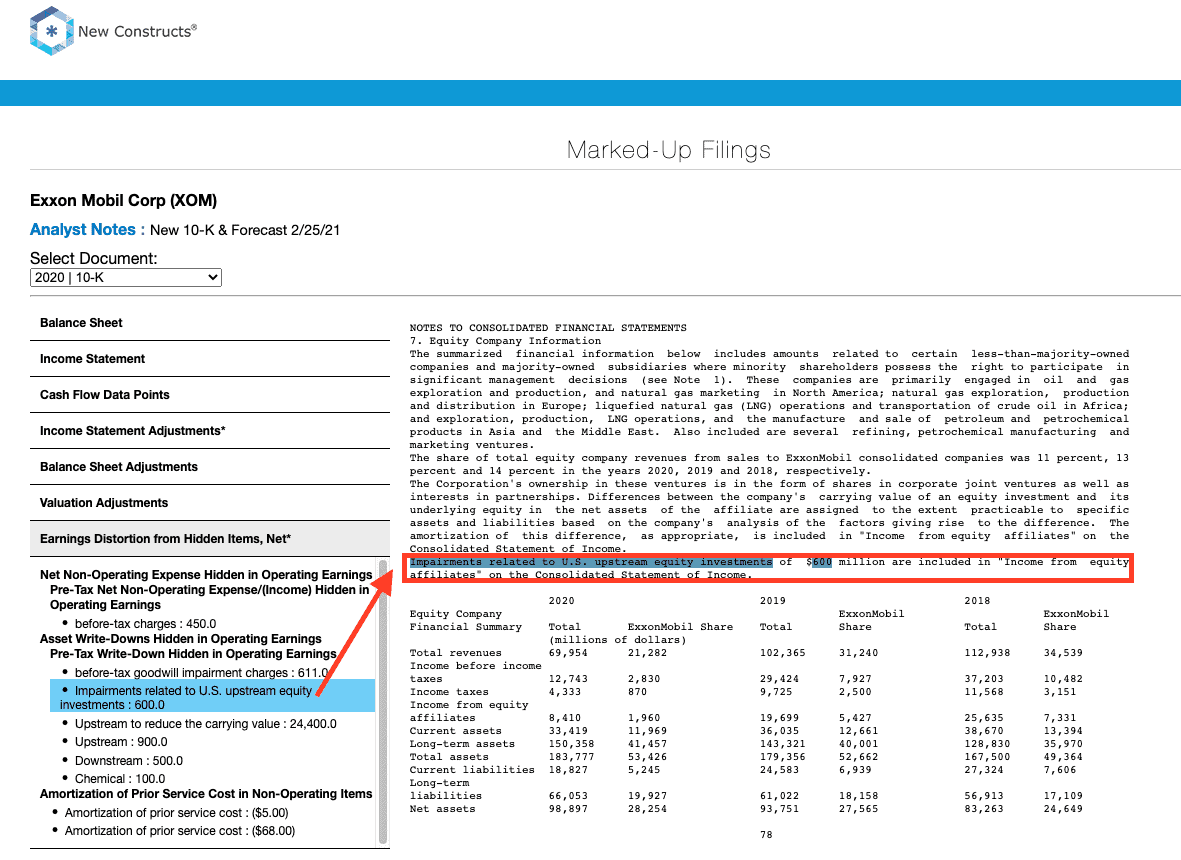The webpage features a stark white background, prominently displaying the title "New Constructs" at the top, followed by a blue horizontal bar. Just below this bar is a section titled "Marked Up Filings," which details various financial documents and data points.

On the left-hand side, the vertical menu lists the following for ExxonMobil Corporation (Ticker: XOM): Analyst notes on the new 10-K report, and a forecast for 2521. It allows selection of various financial documents for the year 2020, including the 10-K report, Balance Sheet, Income Statement, and Cash Flow Data Points. There are also adjustments sections for the Income Statement, Balance Sheet, and Valuation, as well as various earnings distortions and hidden items. Notable entries include:

- **Earnings Distortion from Hidden Items Net:** Pre-tax net non-operating expenses hidden in operating earnings are noted at $450 million.
- **Asset Write-downs:** Pre-tax write-downs, hidden in operating earnings before tax, include:
  - Goodwill Impairment Charges: $611 million
  - U.S. Upstream Equity Investments: $600 million
  - Other Upstream Charges: Various amounts including $24,400 million, $900 million
  - Downstream: $500 million
  - Chemical: $100 million
  - Amortization of Prior Service Cost and Non-operating Items: $5 million and $68 million respectively.

On the right-hand side, there's a detailed segment titled "Notes to Consolidated Financial Statements," specifically Note 7 "Equity Company Information." This section summarizes financial information for less than majority-owned companies and majority-owned subsidiaries where minority shareholders have significant management decision rights. 

Key business operations listed include:
- Oil and gas exploration and production in North America
- Natural gas marketing in Europe
- Liquefied natural gas (LNG) operations and crude oil transportation in Africa
- Exploration, production, LNG operations, and petroleum and petrochemical product manufacture in Asia and the Middle East
- Several refining, petrochemical manufacturing, and marketing ventures

The share of total equity company revenues from sales to ExxonMobil consolidated companies was 11%, 13%, and 14% for the years 2020, 2019, and 2018 respectively. Additionally, a key note mentions impairments related to U.S. upstream equity investments of $600 million, highlighted in red, with a red arrow drawing attention from the section on the left.

Finally, a summary table of equity company financials is presented, showing data in millions of dollars, broken down into ExxonMobil's share versus total amounts over the years 2020, 2019, and 2018:

- **Total Revenues:**
  - 2020: Total $69,954M, ExxonMobil Share $21,282M
  - 2019: Total $102,365M, ExxonMobil Share $31,240M
  - 2018: Total $112,938M, ExxonMobil Share $34,539M
- **Income Before Income Taxes:**
  - 2020: $12,743M, ExxonMobil Share $3,870M
  - 2019: $28,320M, ExxonMobil Share $8,232M
  - 2018: $29,424M, ExxonMobil Share $8,821M
- **Income Taxes:**
  - 2020: $4,333M, ExxonMobil Share $870M
  - 2019: $9,725M, ExxonMobil Share $2,500M
  - 2018: $11,568M, ExxonMobil Share $3,151M
- **Income from Equity Affiliates:**
  - 2020: $8,410M, ExxonMobil Share $1,960M
  - 2019: $19,699M, ExxonMobil Share $5,427M
  - 2018: $25,635M, ExxonMobil Share $7,331M
- **Current Assets:**
  - 2020: $33,419M, ExxonMobil Share $11,969M
  - 2019: $36,035M, ExxonMobil Share $12,661M
  - 2018: $38,670M, ExxonMobil Share $13,394M
- **Long-Term Assets:**
  - 2020: $150,358M, ExxonMobil Share $41,457M
  - 2019: $143,321M, ExxonMobil Share $40,001M
  - 2018: $128,830M, ExxonMobil Share $35,970M
- **Current Liabilities:**
  - 2020: $18,827M, ExxonMobil Share $5,245M
  - 2019: $24,583M, ExxonMobil Share $6,939M
  - 2018: $27,324M, ExxonMobil Share $7,606M
- **Long-Term Liabilities:**
  - 2020: $66,053M, ExxonMobil Share $19,927M
  - 2019: $61,022M, ExxonMobil Share $18,150M
  - 2018: $56,913M, ExxonMobil Share $17,109M
- **Net Assets:**
  - 2020: $98,897M, ExxonMobil Share $28,254M
  - 2019: $93,751M, ExxonMobil Share $27,565M
  - 2018: $83,263M, ExxonMobil Share $24,649M

The page ends with an isolated note stating "$78," which appears unrelated to the preceding content.